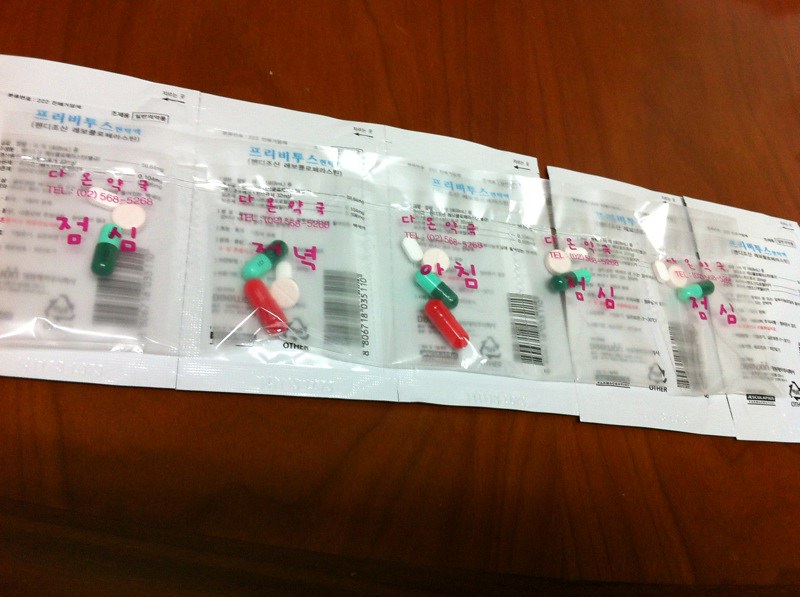The photograph showcases a row of five blister packs of pills, arranged from the upper left corner to the middle right, laid across a dark wooden table. The blister packs are attached to white paper, each displaying a combination of green, dark green, red, and white pills in a clear plastic covering. The green and dark green pills are capsule-shaped, as are the red ones. The white pills include both small oval and circular forms. The white paper backing prominently features purple and blue kanji characters, as well as black writing and a recycling symbol, though the specific text is indistinguishable. A barcode is visible in the lower right corner of the blister packs. The vibrant colors of the pills stand out distinctly against the white background and the dark wooden surface beneath them. The packages extend across the table, partially cut off by the edge of the photograph, highlighting the neatly organized array of this medical prescription.